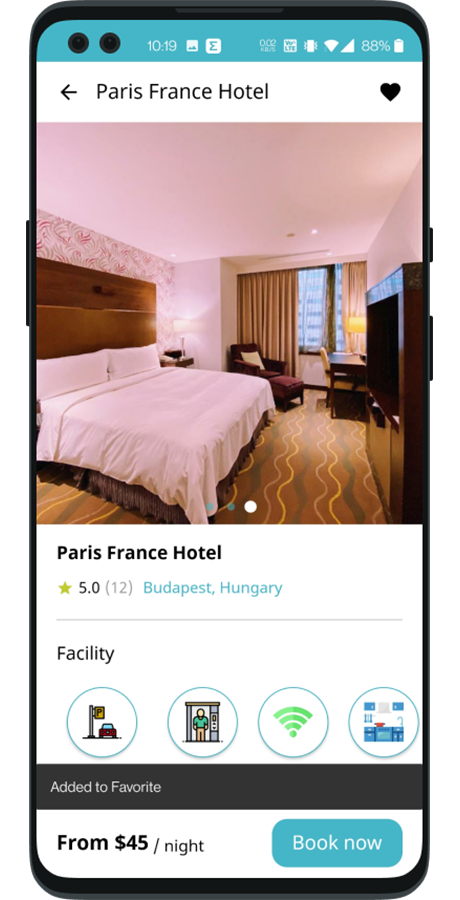This is a cell phone screenshot of a black iPhone displaying a travel search engine page. The website shows a listing for a hotel in Paris, France. At the top of the screen, there's a back arrow on the left and a heart icon on the right, indicating options to go back or save the listing. 

The hotel listing features prominently in the center, indicating it's a highly-rated 5-star hotel based on 12 votes. Below the hotel information, the text "Budapest, Hungary" is displayed in light blue letters, possibly referring to other recommended destinations.

A section labeled "Facility" follows, showcasing four circular icons representing the hotel's amenities: a car and flag (likely indicating parking and flags for multilingual support), a person at a vending machine, Wi-Fi, and photos.

At the bottom left of the screen, the price is listed as starting from $45 a night. To the right, a prominent blue "Book Now" bar allows potential guests to quickly make a reservation.